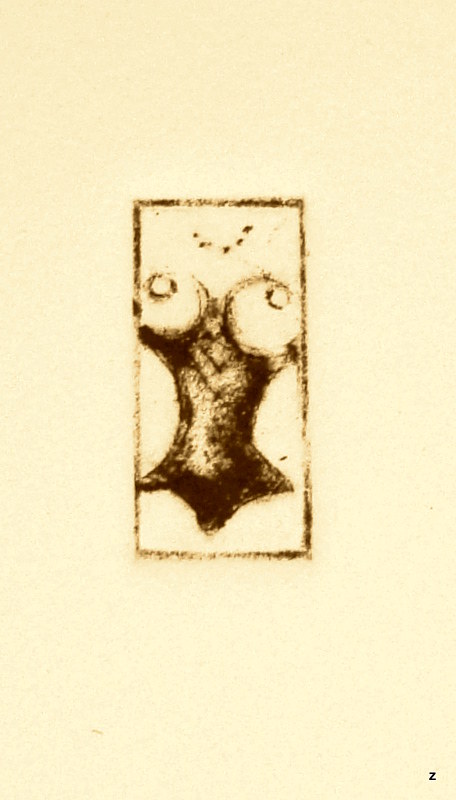The image is of a detailed, black-and-white drawing on aged, ivory-colored paper with a visibly textured, grainy appearance. The focal point of the illustration is a stylized, hourglass-shaped figure of a woman's chest and waist, framed within a vertical rectangle. The woman, viewed from the neck down, is depicted wearing a tight-fitting, black bustier or corset which cinches her waist uncomfortably, emphasizing her hips and chest. Around her neck, a delicate necklace, possibly pearls, is partially visible. The lines of the drawing are rough and pencil-like, giving it a sketchy, yet detailed texture. The background remains a stark, ivory color, further highlighting the contrast of the woman's form in the center. At the bottom right of the illustration, a small, dark "Z" is faintly noticeable.